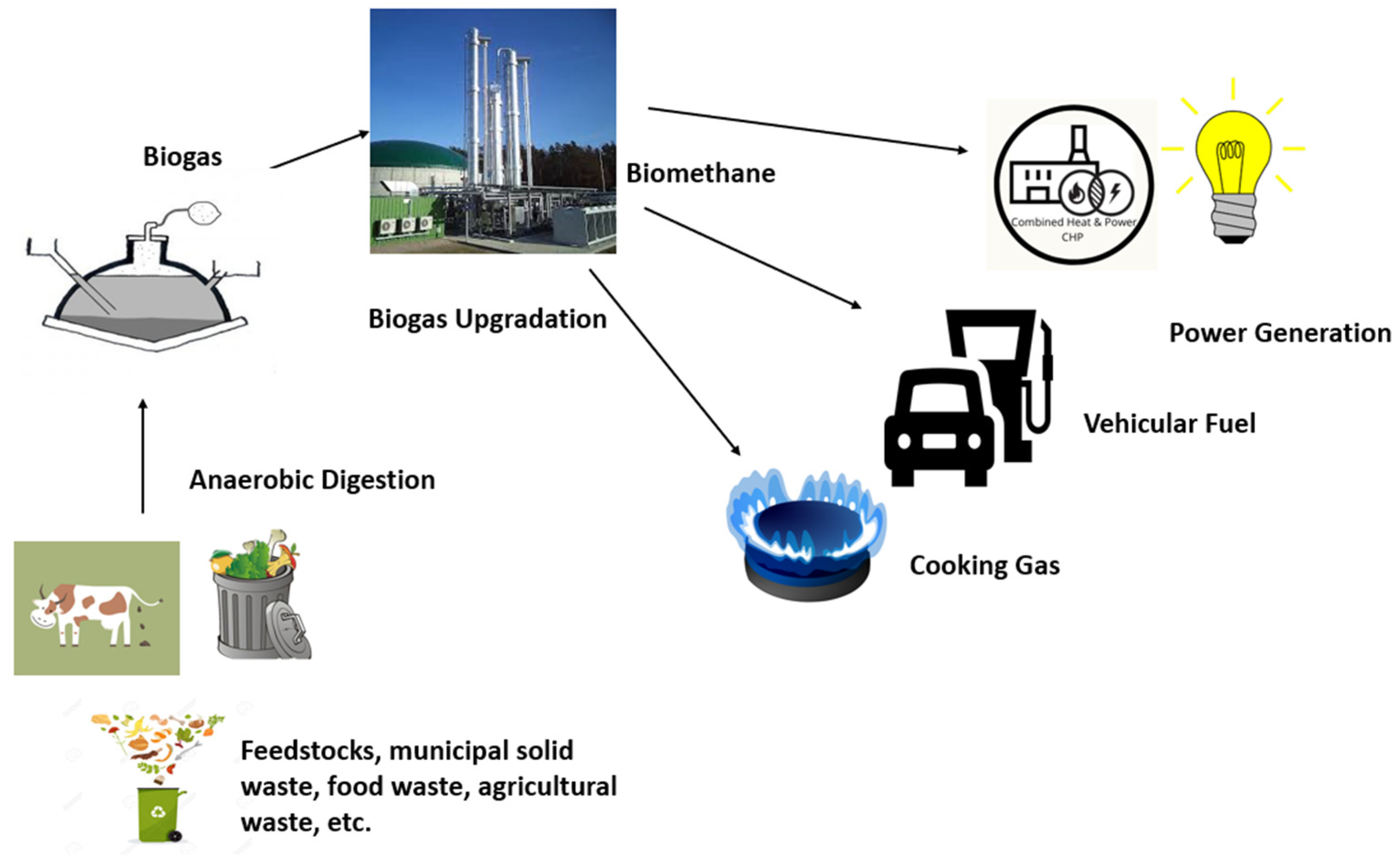This detailed diagram illustrates the biogas production and utilization process. At the bottom left, a labeled recycling bin holds various feedstocks such as municipal solid waste, food waste, and agricultural waste. Above it, a cartoon cow is depicted defecating. To the right, an open trash can overflow with waste, all labeled as "Anaerobic Digestion," the process converting these wastes into biogas.

The biogas is shown stored in a dome-shaped container with a spout on top and two smaller diagonal spouts on the sides, with a V-shape at the bottom, labeled "Biogas." An arrow points from this biogas container to an industrial facility labeled "Biogas Upgradation," which features several smokestacks and a small green section with white parts.

From this facility, three arrows emerge: one leads to a burner emitting a blue flame labeled "Cooking Gas"; another to a gas pump symbol overlapping a car labeled "Vehicular Fuel"; the third arrow heads to a building symbol, encircled by overlapping icons of a flame and a lightning bolt, representing a power plant. Beside this building, a lit light bulb is labeled "Power Generation," indicating the use of biomethane for electricity production.